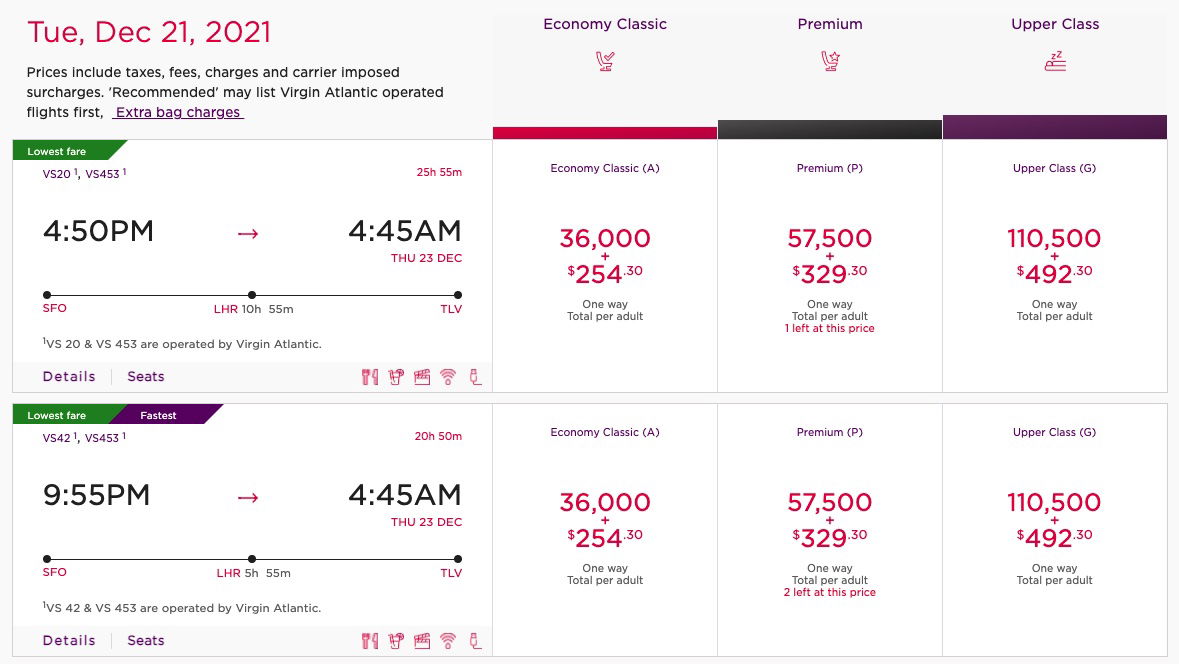Screenshot Description for Flight Comparison Website

This cropped desktop screenshot displays a travel booking website for flight arrangements on Tuesday, December 21st, 2021. The date is highlighted in a pinkish-red font. In black text, it indicates that prices include taxes, fees, charges, and carrier-imposed surcharges. The recommended mailing list version prioritizes Atlantic-operated flights. An extra bag charge option is available as a clickable purple link.

On the right side, there is a list of cabin classes: Economy Classic, Premium, and Upper Class, each in purple text. Economy Classic is depicted with an airplane chair icon, Premium with an airplane chair icon paired with a star, and Upper Class with an icon of a person lying down, symbolizing a sleeping position. These classes are further highlighted by color bars: hot pink for Economy Classic, black for Premium, and purple for Upper Class.

The lowest fare, highlighted in green, outlines a travel route from San Francisco International Airport (SFO) to Tel Aviv's Ben Gurion Airport (TLV) with a layover in London's Heathrow Airport (LHR). The total travel time is 10 hours and 55 minutes.

Details for the first flight include:
- Departure from SFO at 4:50 p.m.
- Arrival at LHR at 4:45 a.m. on December 23rd. 
The flight amenities listed are meal service, drinks, in-flight entertainment, Wi-Fi, and device plug-ins. The screenshot does not display the currency for the prices.

The flight options have identical pricing:
- Economy Class: 36,000 points + $254.30 (one way per adult)
- Premium: 57,500 points + $329.30 (one way per adult, with only one seat remaining at this price)
- Upper Class: 110,500 points + $492.30 (one way per adult)

The second flight option, marked as the lowest fare and also the fastest, departs at 9:55 p.m. with a 5-hour and 55-minute layover, arriving at 4:45 a.m. It includes the same amenities as the first flight option. The prices remain consistent with the first flight option, with two seats left at this price.

In summary, the screenshot compares flights from San Francisco to Tel Aviv via London on December 21st, 2021, highlighting various cabin classes and identical fares, leaving the user to decide based on layover durations and departure times.